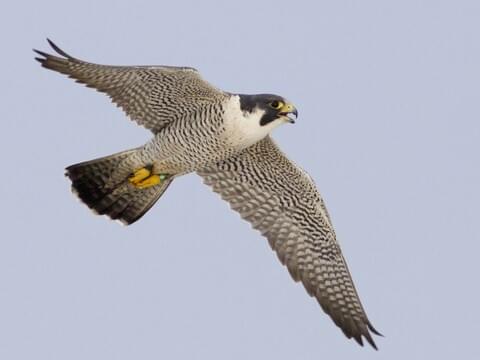This is a detailed color photograph of a peregrine falcon in mid-flight, prominently occupying the frame and flying towards the right. The bird's iconic features are clearly visible from an underside perspective. It boasts a dark black hood on its head, complemented by a short, hooked yellow beak and dark black eyes, encircled by a white ring behind its head. Its wings are fully outstretched, showcasing a striking pattern of white, brown, and black feathers, aiding its camouflage in the skies. The falcon's body is adorned with a peregrine plume pattern, blending whites with various browns and grays. Its feet, colored in a distinct yellow-orange hue, are pulled up underneath its body, and one foot is marked with a tracking band, possibly indicating it was once monitored or cared for in captivity. The tail feathers exhibit a gradient from dark brown to dark gray. The sky behind the falcon transitions from dark gray to light gray, suggesting an overcast day. There are no other entities or structures in the background, emphasizing the solitary splendor of the falcon in this descriptive photograph.